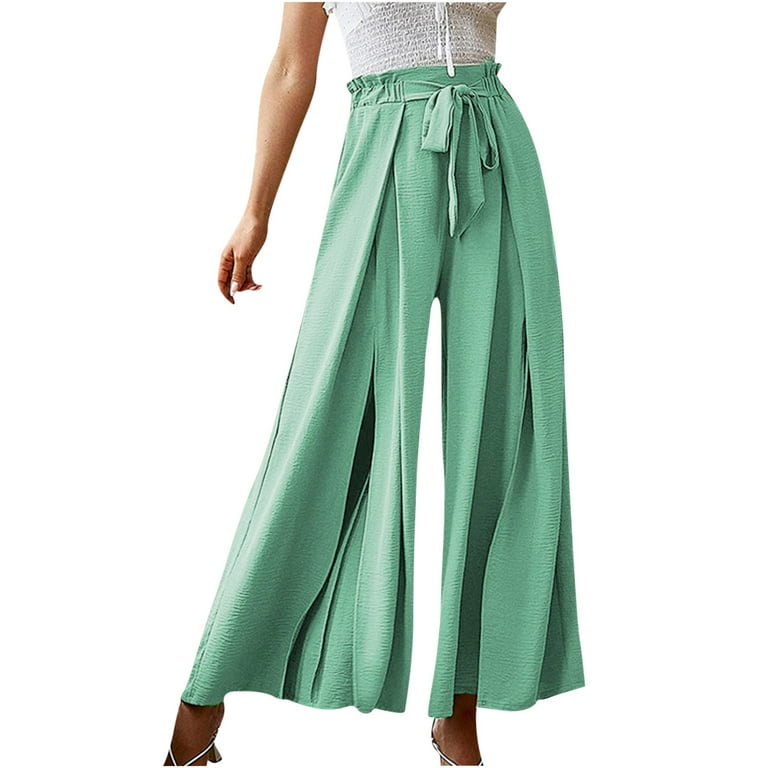The image depicts the bottom half of a woman standing against a white background, showcasing her attire. She is dressed in flowing, wide-leg green pants that cinch at the waist with a tie. The fabric of the pants gives them a resemblance to a long skirt due to their billowy nature. The woman is also wearing a white top, though only the lower portion of the top is visible, with a ribbon or tie detail hanging from it. Her left arm is extended downward, and her hand is slightly curled. The lower part of her legs is visible, revealing the tops of her feet and ankles adorned with white strapped shoes. The overall focus of the photograph seems to be on her green pants, which are the central element of the outfit. This composition suggests that the image may be intended to highlight these clothing items, possibly for an advertisement or fashion feature.